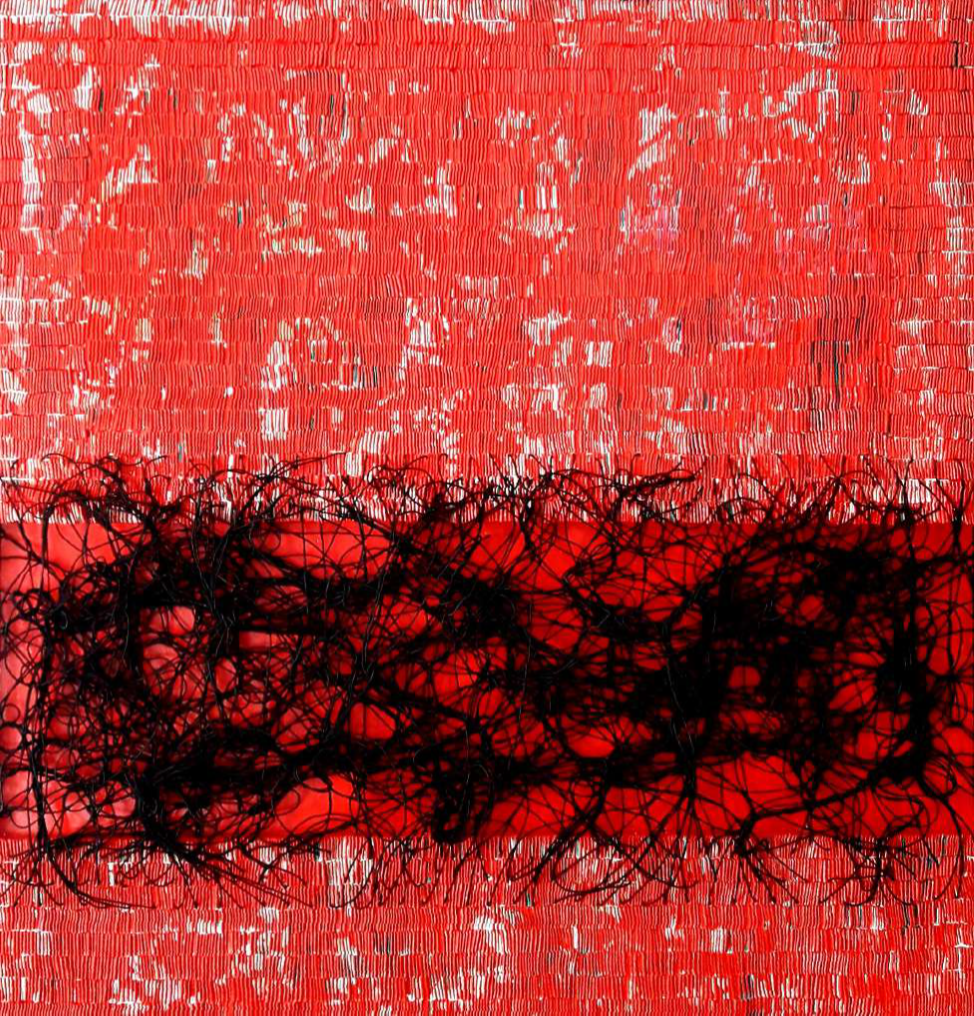The image under discussion appears to be an intricate modern artwork, potentially a painting or collage, alternating between delicate nuances and bold impositions. The main composition showcases a semi-transparent red background reminiscent of magnified curtain shears, woven with white or gray elements that form squarish or rectangular patterns, lending the piece a sense of stitched texture. Dark smudges intermingle with clearer spaces, creating variable depth and visual interest. Dominating the lower portion, but not fully covering it, a solid, thick red ribbon spans from one-eighth to three-eighth up the image. This ribbon is accentuated by erratic black threads resembling strands of hair, sprawled across in random, web-like forms, adding an element of chaotic intrigue. These black threads intensify the dynamism of the piece while the background retains a more measured, grid-like pattern in red and white. The entire composition is devoid of text, emphasizing its role as a purely artistic creation meant to provoke thought and interpretation.